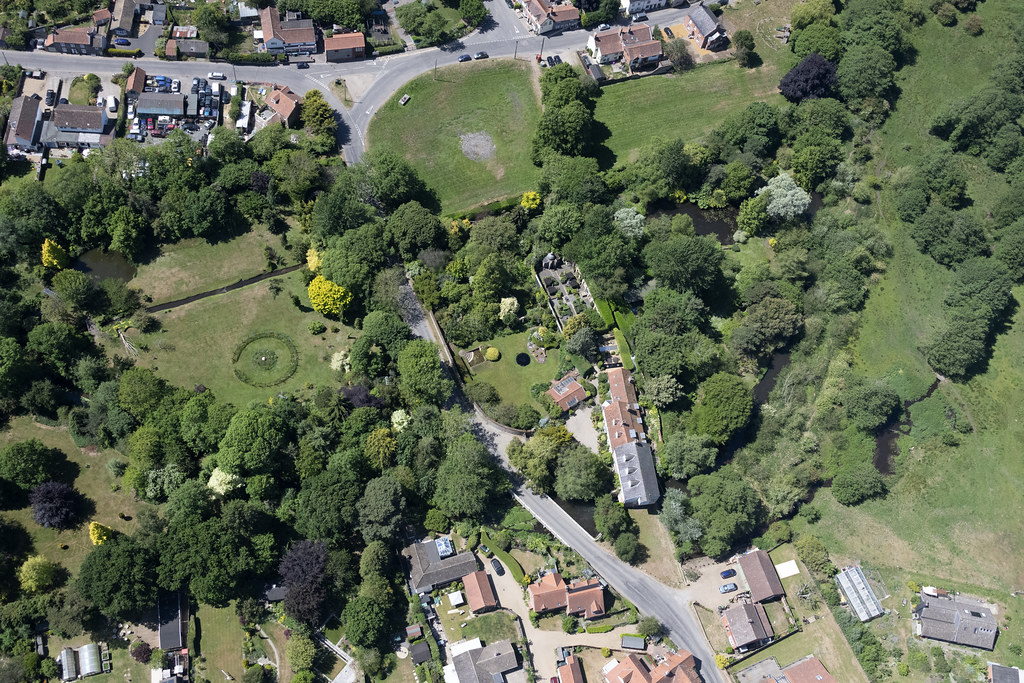The image is a high-resolution, top-down aerial view of a town or two interconnected neighborhoods, likely taken from a drone or an airplane. The photo predominantly features a winding road that begins in the top left corner and snakes its way towards the bottom right. The landscape is dotted with numerous houses, prominently seen through their rooftops, and is lush with trees and greenery, creating a forested appearance. The road intersects in a Y-shape towards the bottom, giving paths to the right and left. In the top left portion, the area appears more developed with some businesses indicated by an accumulation of cars, suggesting a shop or gas station. A significant grassy field runs through the central area of the photo, which also features a round landscaped ring. No people are visible in the image, but several cars can be seen on the roads. There appears to be a separation in the lawn, possibly a trail or stream, delineating property lines and adding to the picturesque, verdant setting of the residential area.